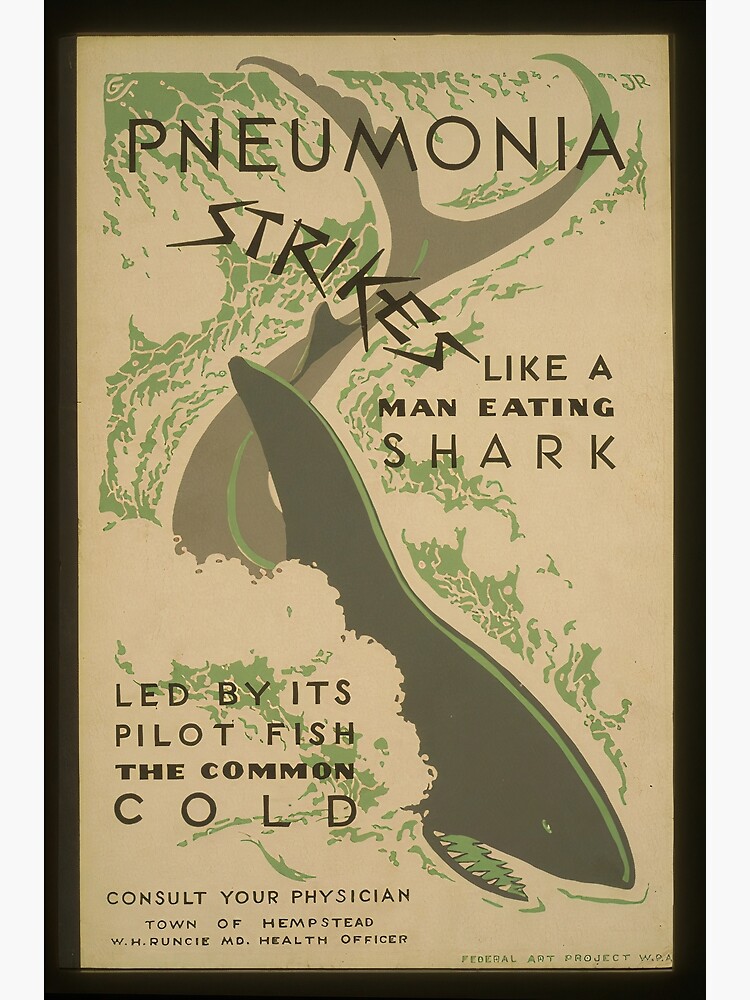The image is an advertisement flyer for a public health program with a vividly designed tan background adorned with green areas. Dominating the center is a menacing gray shark outlined in green, with a green mouth and sharp white teeth, resembling a predatory force traveling at high speed. The design cleverly integrates elements that mimic a highway or road, with the shark's tail forming twin ends that resemble converging streets, and a green band that looks like traffic signaling.

At the top of the flyer, bold black text reads, "Pneumonia strikes like a man-eating shark," emphasizing the danger of the disease. Below it, another line states, "led by its pilot fish, the common cold," highlighting the common cold as a precursor. On the bottom left next to the shark, in smaller black text, it advises, "consult your physician." Further details include, “Town of Hempstead W.H. Runch C.M.D. Health Officer.” In the very bottom right, light green text signifies the "Federal Art Project," suggesting the flyer was part of a larger public health art initiative.